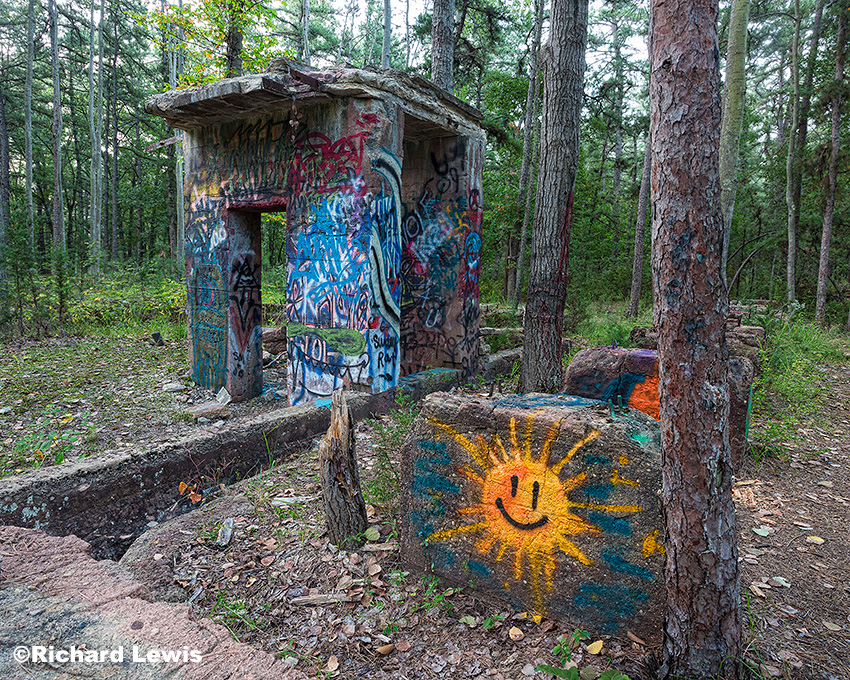The image depicts a forest setting featuring the remnants of an old shack or shelter. The central focus is a graffiti-covered structure, slightly left of center, which appears to be made of wood. The shack has a cube-like shape, taller than it is wide, and includes two notable openings: a large one on the right and a smaller one on the left. The flat roof is composed of wooden planks, and where doors once existed, there are now empty frames allowing a view straight through the structure.

Surrounding this central structure are several concrete blocks and remnants of walls, adorned with extensive graffiti in an array of colors including blue, gold, black, red, green, yellow, gray, and brown. A prominent feature among the graffiti is a black smiley face on one of the concrete blocks positioned towards the bottom right of the image.

Trees populate the scene, both to the right of the structure and in the background, enhancing the forest atmosphere. Below the structures, the forest floor is visible, covered with leaves and debris. The entire scene is marked by the sense of abandonment and defacement, accentuated by the vivid graffiti.

In the bottom left-hand corner of the photograph, the text "Copyright Richard Lewis" is visible in white font, asserting the ownership of the image.